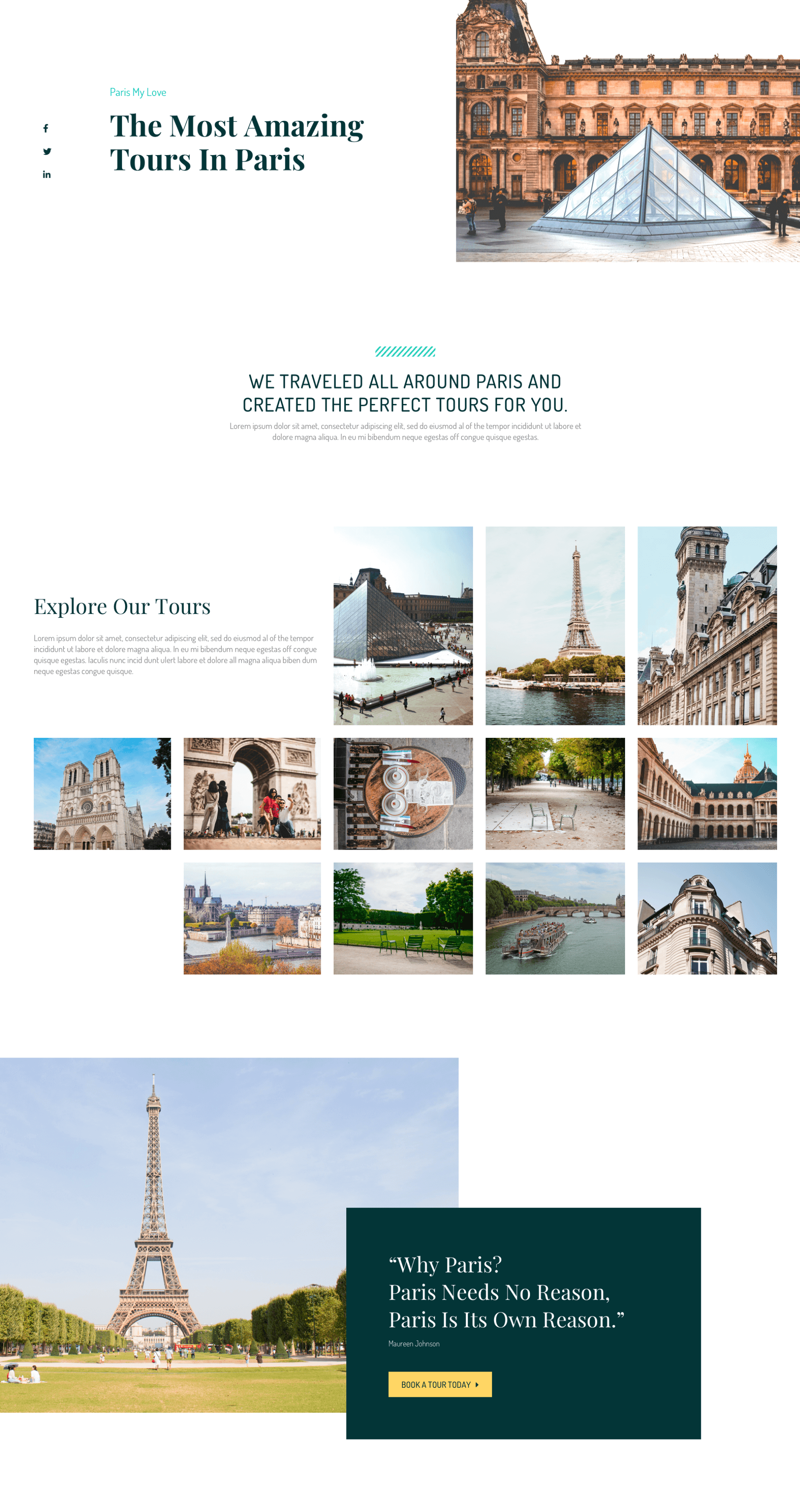Here is a refined and detailed caption for the image:

This is a screenshot of an informative webpage dedicated to promoting tourism in Paris. The page features numerous links to exceptional tours throughout the city, emphasizing the vast exploration opportunities available. Prominent quotes such as, "Why Paris? Paris needs no reason. Paris is its own reason," underscore the allure of the city. Accompanying the text are captivating images, including iconic landmarks like the Eiffel Tower, the Louvre, and serene scenes of the Seine River with a boat cruising on it. The overall design of the webpage boasts a clean, white background with strategically placed photographs that add visual appeal. Interactive elements include clickable photos under the section "Explore Our Tours," which likely direct users to specific tour options. At the bottom of the page, a conspicuous yellow box invites visitors to "book a tour today," providing immediate access to tour reservations. The webpage assures potential tourists of expertly curated tours, crafted by individuals with extensive experience exploring various parts of Paris, ensuring top-notch quality and memorable experiences.